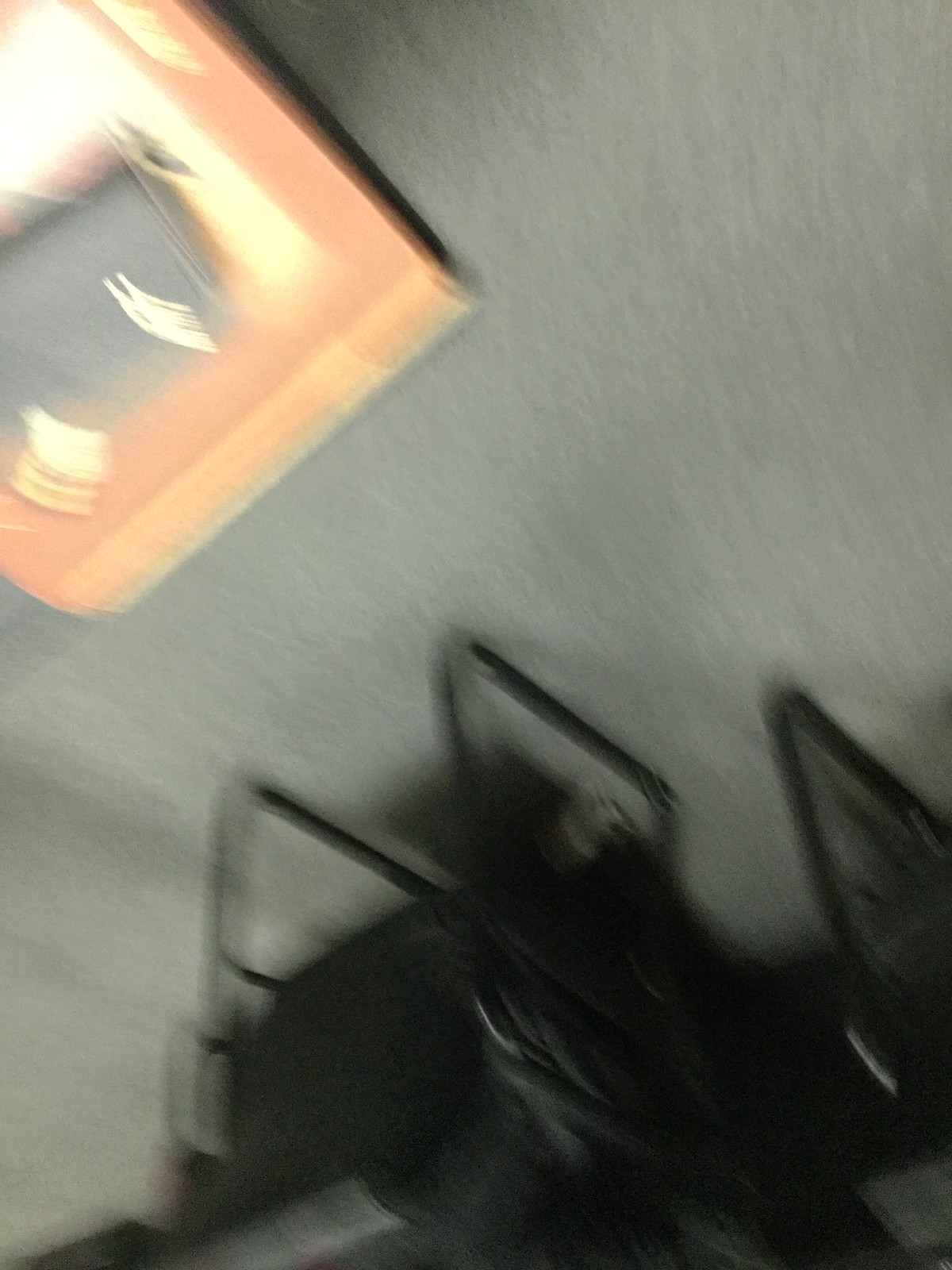The image depicts a blurry and out-of-focus scene, likely taken inadvertently. The primary focus is on a gray carpeted floor. In the top left corner, there is a thin rectangular cardboard box with its bottom flap slightly open, facing downward. On top of this box rests an indistinct gray object, highlighted by streaks of light. Towards the bottom of the frame, there is a black chair with a padded back and a sturdy frame, resembling those commonly found in waiting rooms. The image, captured in portrait mode, provides minimal discernible context, suggesting it might have been an accidental photograph.